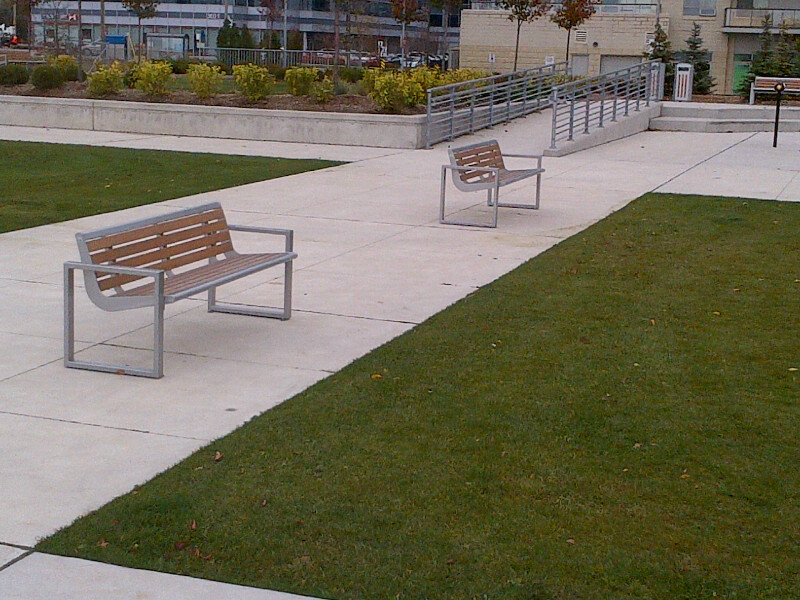The image features an expansive outdoor area, possibly a college campus or a new office complex. The focal point is two empty park benches made of gray metal with dark brown wooden slats, positioned on a wide, light gray concrete walkway. This walkway is bordered by meticulously maintained green grass in square or rectangular patches. 

In the area surrounding the benches, the pathway provides ample room for pedestrian traffic, with sections leading to various areas. To the right of the benches lies a handicap ramp with steel railings, leading to an elevated cement platform, flanked by a set of two concrete steps. Here, another matching bench and a silver and brown trash can are visible. 

In the distant background, there are manicured, low-lying yellow and green shrubs and young trees with thin trunks and small clusters of leaves. Additionally, there are small evergreen trees suggesting the landscaping is relatively new, likely within the past decade. 

The backdrop of the image features beige and light brown brick buildings on the right, with designated parking spaces, and on the left, a larger gray concrete and glass building, reflecting a more modern architectural style. The overall feel of the area is open, clean, and well-organized, indicative of a newly developed or well-maintained urban or institutional environment.